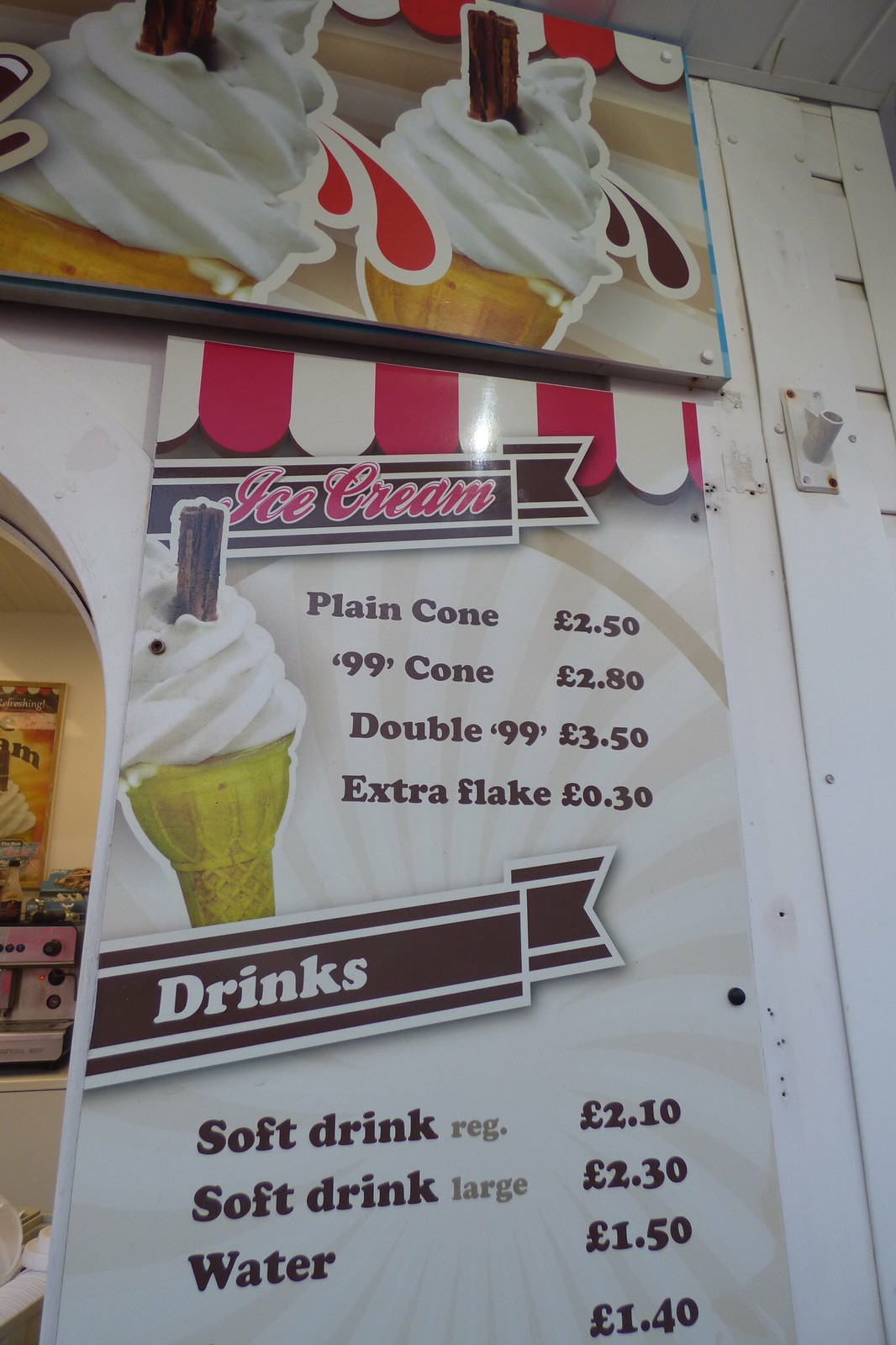This color photograph, taken in portrait orientation, captures the exterior facade of an ice cream shop. Dominating the center of the image is a vertical menu mounted on the right-hand side of a white wall, adorned at the top with a red and white canopy design. Above the menu, there's a partially visible horizontal banner depicting two soft-serve ice cream cones with churros protruding from the top. The upper-left background features an archway leading into the shop, where a coffee machine and cups are faintly visible. 

The menu is divided into two sections: "Ice Cream" and "Drinks." The ice cream section, under a black banner with pink script reading "Ice Cream," lists options such as Plain Cone ($2.50), 99 Cone ($2.80), Double 99 ($3.50), and Extra Flake ($0.30), accompanied by a photograph of a soft-serve cone with a churro. Below this, another black banner with white text reading "Drinks" details the drink options: Soft Drink Regular ($2.10), Soft Drink Large ($2.30), Water ($1.50), and an unspecified item priced at $1.40. A flagpole without a flag is visible near the menu, contributing to the realistic and detailed depiction of the setting.